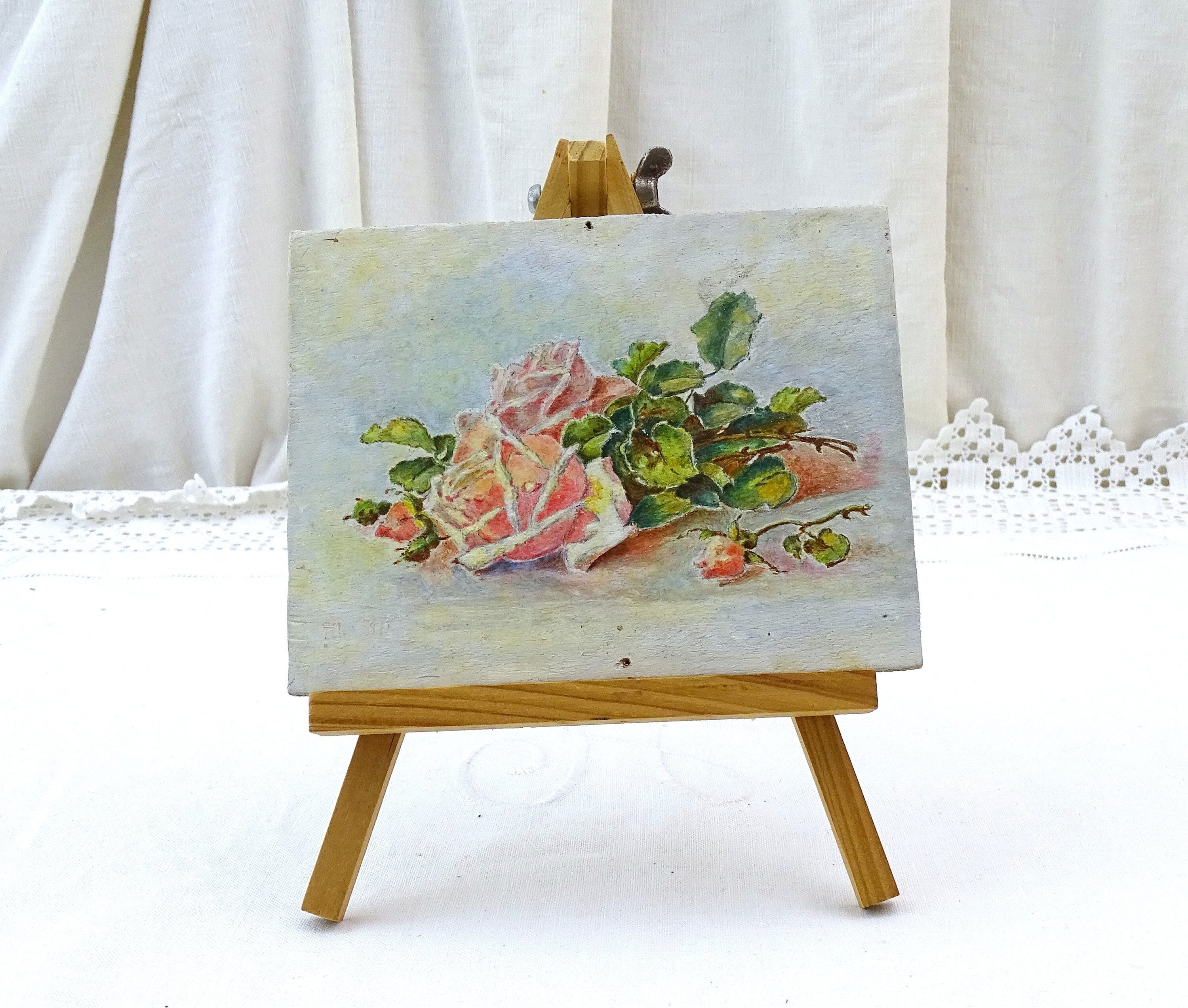The image captures a detailed photograph of a small painting displayed on a light wooden easel, which is placed atop a white tablecloth with a lace edge. The background consists of a white sheet or curtain, adding a soft, delicate ambiance to the scene. The painting itself, a watercolor illustration, features two pink roses with green stems lying horizontally on a faded pale blue background. The roses, accented with white trim, appear as if they are part of a fallen bouquet. This charming composition is elegantly framed by the intricately laced tablecloth and the simple, yet sophisticated, draped background.